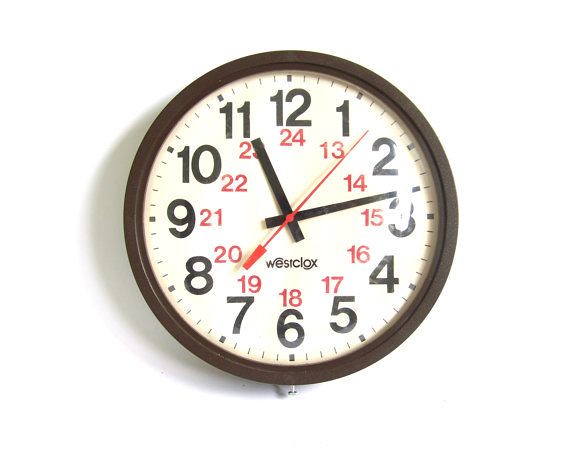This photograph features a standard wall clock with a dark brown or black rim and a white clock face. The clock displays large black numerals from 1 to 12 around its circumference and smaller red numerals from 13 to 24 positioned adjacently for a 24-hour format. Each black numeral is accompanied by minute markers, with bold marks every five minutes. The clock has three hands: the hour and minute hands are black, while the second hand is red and currently pointing between the 1 and 2-second marks. The time displayed is approximately 11:13, though it is unclear whether it is a.m. or p.m. Positioned just below the center of the clock, it bears the logo "Westclox." The clock is mounted on a white wall with visible shadowing on the left side.